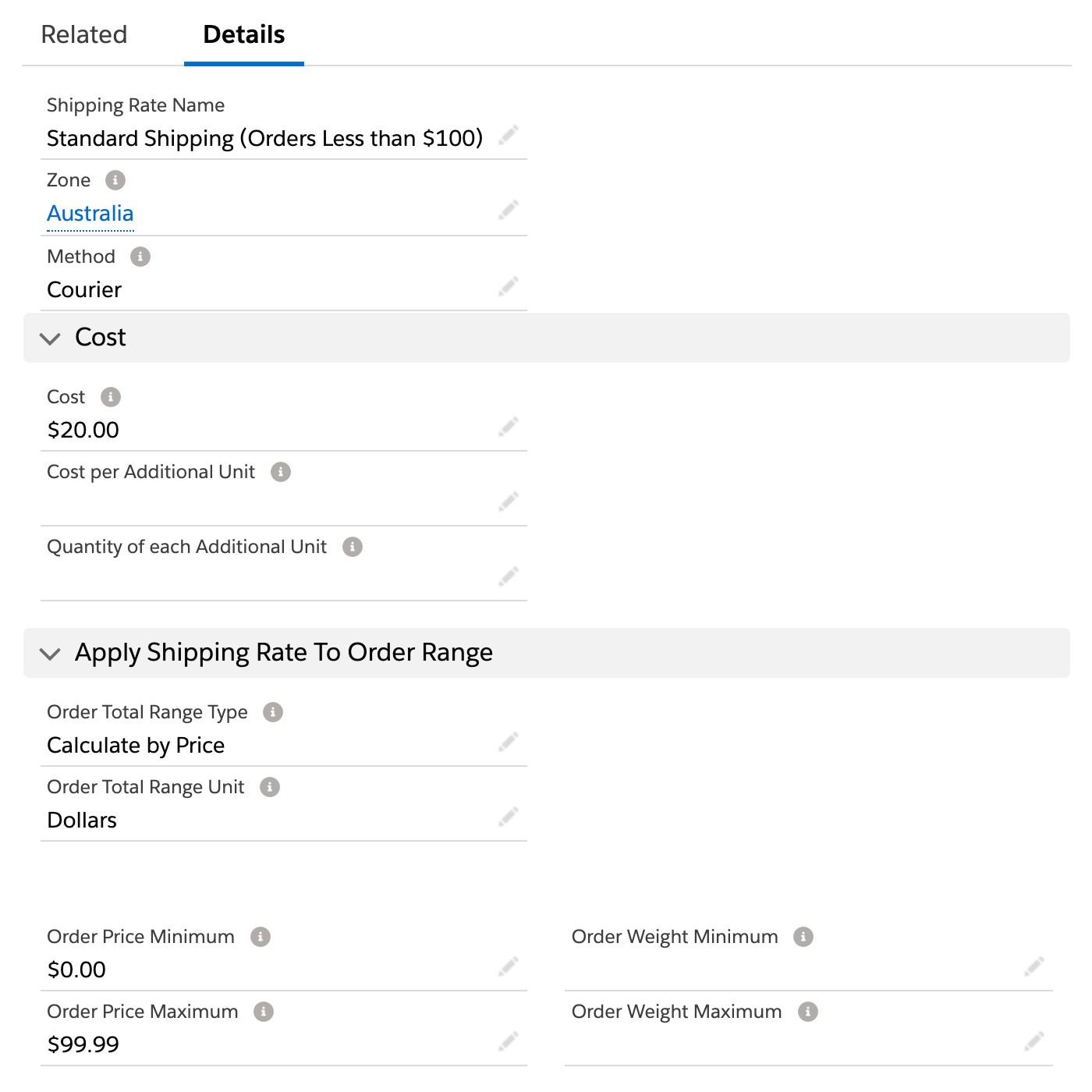The image depicts a detailed interface of a shipping rate configuration page on a white background, structured in a long, rectangular format. 

In the upper left corner, two tabs are visible: the first tab on the left is dark gray and labeled "Related," while beside it, a tab with black text labeled "Details" is highlighted with a blue underline, indicating the current view. 

Below the tabs, there is light gray text reading "Shipping Rate Name." Beneath this, a search bar displays black text stating "Standing Shipping (Orders Less Than $100)," accompanied by a light gray pencil icon on the right, signifying an edit option. 

Further down, the section labeled "Zone" is presented with blue text indicating "Australia." Under "Method," the black text shows "Courier."

Following these sections, a long, horizontal, light gray box appears. Inside, on the left side, is black text labeled "Cost" with a downward arrow next to it. Directly below this, the word "Cost" is repeated in a smaller font, and beneath that, the number "$20" is displayed in black text.

Additional fields below include "Cost Per Additional Unit" and "Quantity of Each Additional Unit," both of which are currently empty.

Another light gray box below contains black text reading "Apply Shipping Rate to Order Range." Absent adjacent text describes parameters like "Order Total Range Type" with "Calculate by Price" below it, and "Order Total Range Unit" with "dollars" listed underneath.

At the very bottom, on the left side, it displays "Order Price Minimum" with "$0" beneath, followed by "Order Price Maximum" marked as "$99.99." On the bottom right, similar fields for "Order Weight Minimum" and "Order Weight Maximum" are shown, both presently blank.